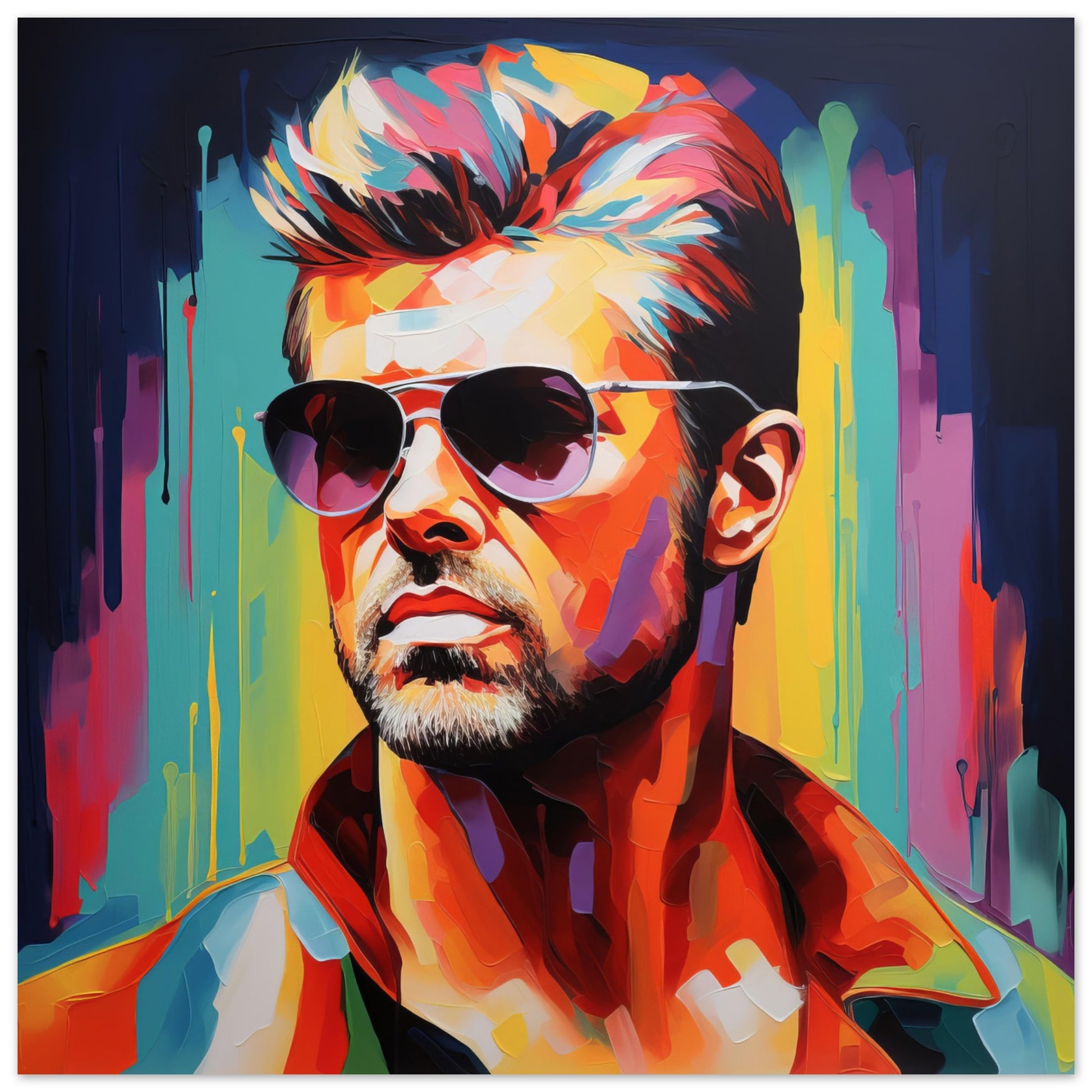This highly stylized, computer-generated painting features a male figure depicted from the shoulders upward. The man wears a tall-collared jacket exhibiting a gradient from vibrant orange to green, white, and blue. His beard and mustache are meticulously painted in black and white. Notably, the man sports silver-framed aviator sunglasses with purple lenses, partially concealing his serious, contemplative expression. His hair, swept up and appearing to be styled with gel, is rendered in striking shades of blue, purple, pink, and yellow. The background complements this colorful palette, blending splotches of blue, yellow, pink, and red with predominantly black corners at the top edges. Despite the vivid and somewhat abstract use of color, the composition achieves a harmonious and engaging visual effect, focusing solely on the man's upper visage without any text or additional context.